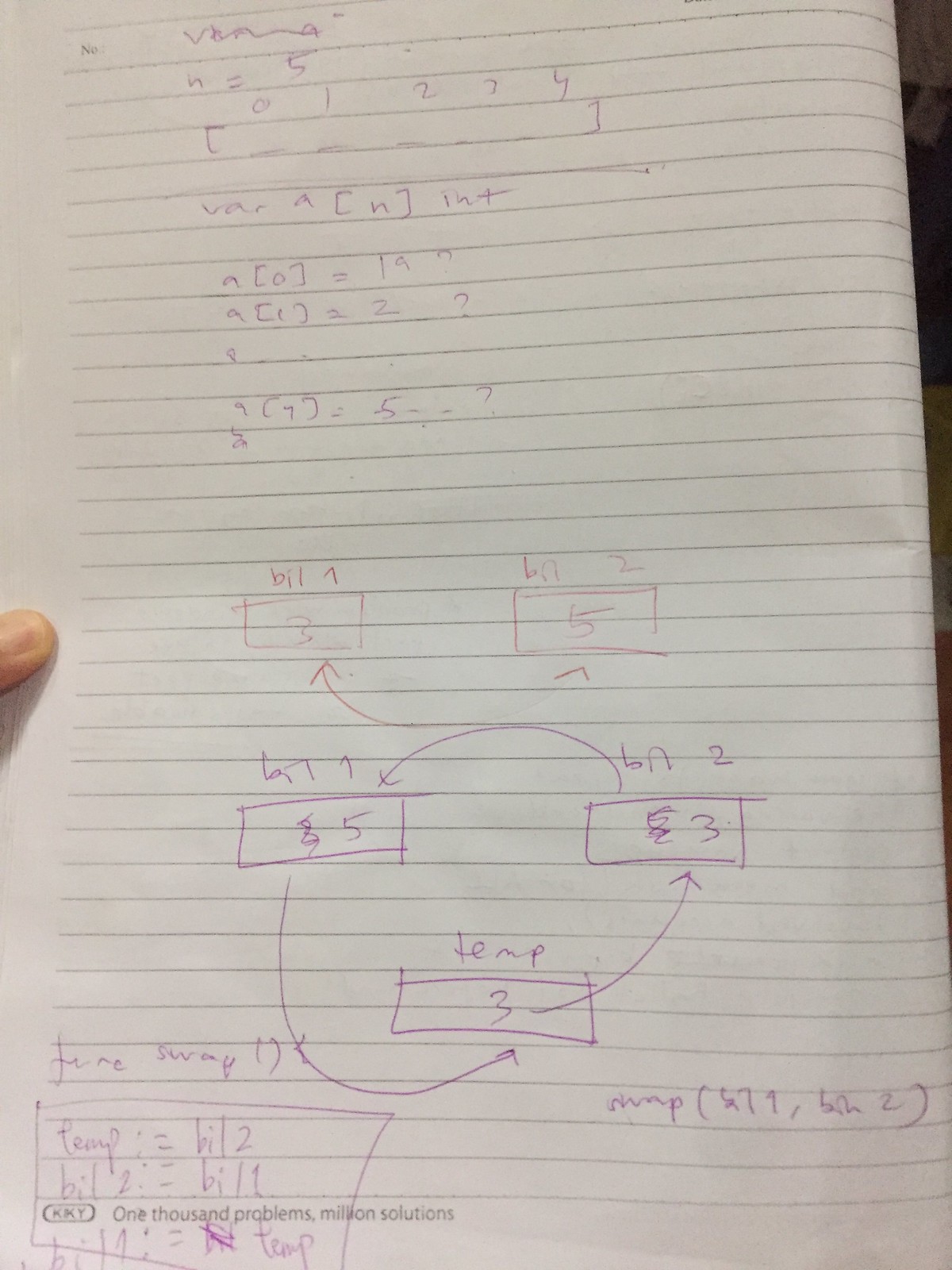This photograph captures a lined piece of paper set against a black background, with part of the background visible on the right side. The paper, displaying neat horizontal lines, features a printed "O" in the upper left corner. The handwriting on the paper, potentially in black ink or pencil, is filled with various numbers and symbols indicative of mathematical or programming notes.

The content begins with "N" followed by "N = 5" and a sequence of numbers "0, 1, 2, 3, 4" accompanied by brackets. It continues with the notation "VARA[N] INT." Below this is the line "A[0] = 1," possibly followed by "19?" and "A[C] 2-2?" 

Further down, there is "7[ ] = 5-?" followed by two rectangles containing the numbers "3" and "5." Beneath these, curved lines with arrows connect to two other rectangles labeled "5" and "3." Below this is another rectangle linked by more curved lines and arrows, with the word "TEMP" situated above a rectangle numbered "3."

The lower section of the paper appears more complex, possibly stating "TEMP = BIL2," "BIL2 = BIL1," and something like "BIL[...] = TEMP." Additionally, the paper includes an oval printed with the letters "KKY" and the motivational phrase, "One Thousand Problems, Million Solutions."